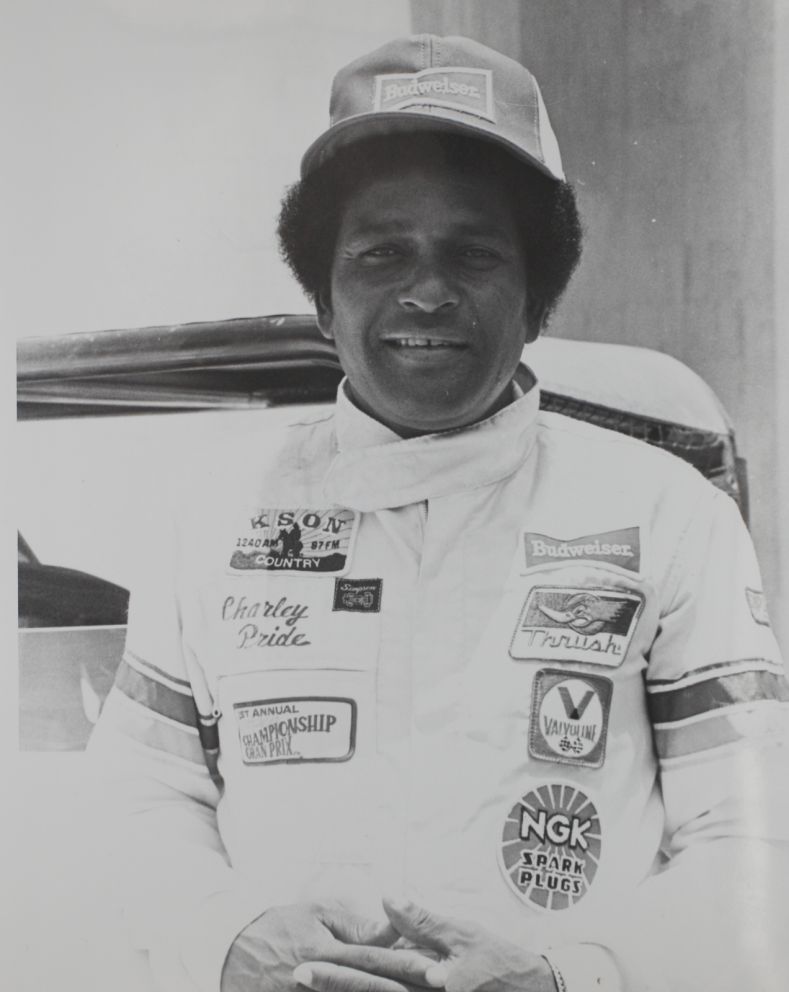The black and white photograph features an African American man, identified as Charlie Pride, standing and posing for the camera. He has a round afro partially covered by a baseball cap with a prominent Budweiser patch. Charlie is dressed in a white racing jumpsuit adorned with numerous sponsor patches, including Budweiser on his chest, Valvoline with its characteristic "V," NGK Spark Plugs, and several others. His name, "Charlie Pride," is embroidered in cursive on the right side of his jumpsuit. With his hands folded in front of him and a gentle smile revealing some of his teeth, he stands in front of an indistinct light-colored object, possibly part of a car. This image might date back several years, adding a layer of historical interest to the scene.